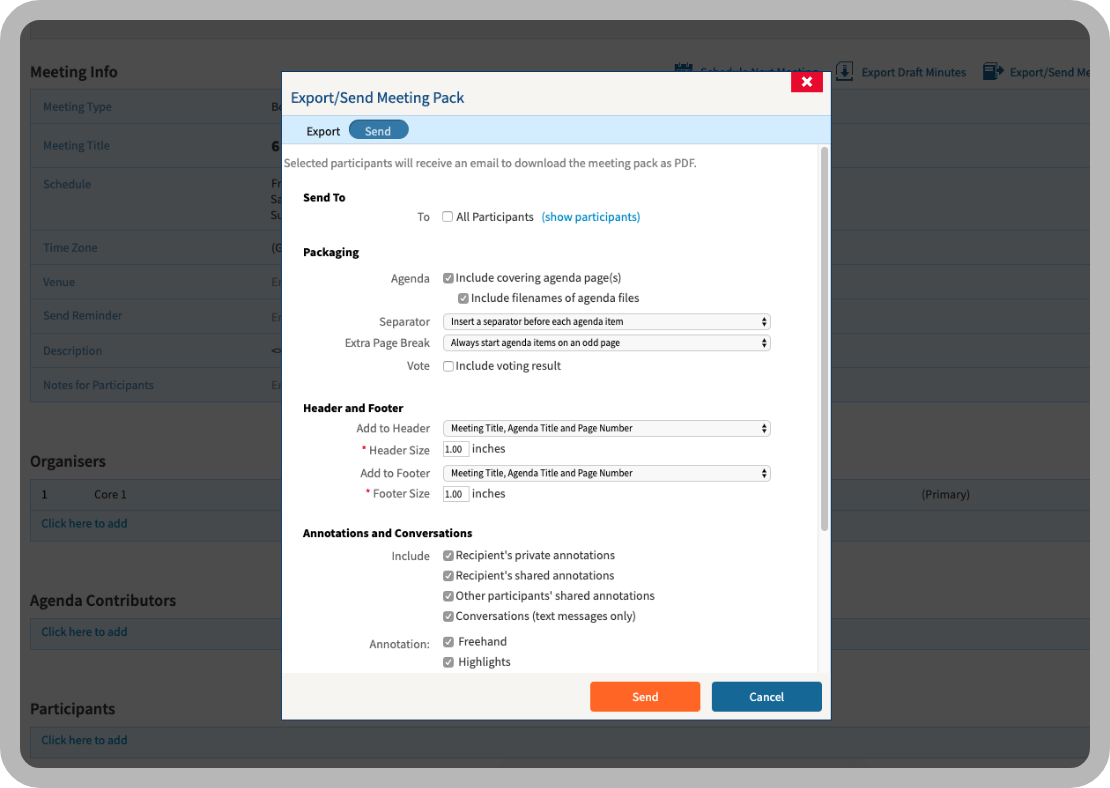The image displays a user interface for exporting and sending a meeting pack. The options available include:

- **Text Categories:**
  - **Export, Send Meeting Pack:** Allows users to send the meeting pack to selected participants via email as a PDF.
  - **Send to All Participants:** An option to distribute the meeting pack to all participants.
  - **Show Participants:** Displays a list of participants involved in the meeting.
  - **Packaging:** Options around organizing and formatting the meeting pack.
  - **Agenda:** Options relevant to the agenda including:
    - **Include Covering Agenda Pages:** Adds cover pages to the agenda.
    - **Include File Names of Agenda Files:** Ensures file names appear on the agenda.
    - **Separator:** Inserts a separator before each agenda item.
    - **Extra Page Break:** Ensures agenda items start on an old (new) page.
  - **Vote:** Option to include voting results in the meeting pack.
  - **Header and Footer:** Customizations including:
    - **Add to Header:** Meeting title, agenda title, and page number.
    - **Header Size:** Adjustable, specified as 1 inch in the example.
    - **Add to Footer:** Reiteration of meeting title, agenda title, and page number.
    - **Footer Size:** Also adjustable, set to 1 inch.
  - **Annotations and Conversations:** Includes:
    - **Private and Shared Annotations:** Recipients' private and shared annotations.
    - **Conversations:** Text messages and highlights among participants.

Prominently displayed action buttons include "Send" and "Cancel."